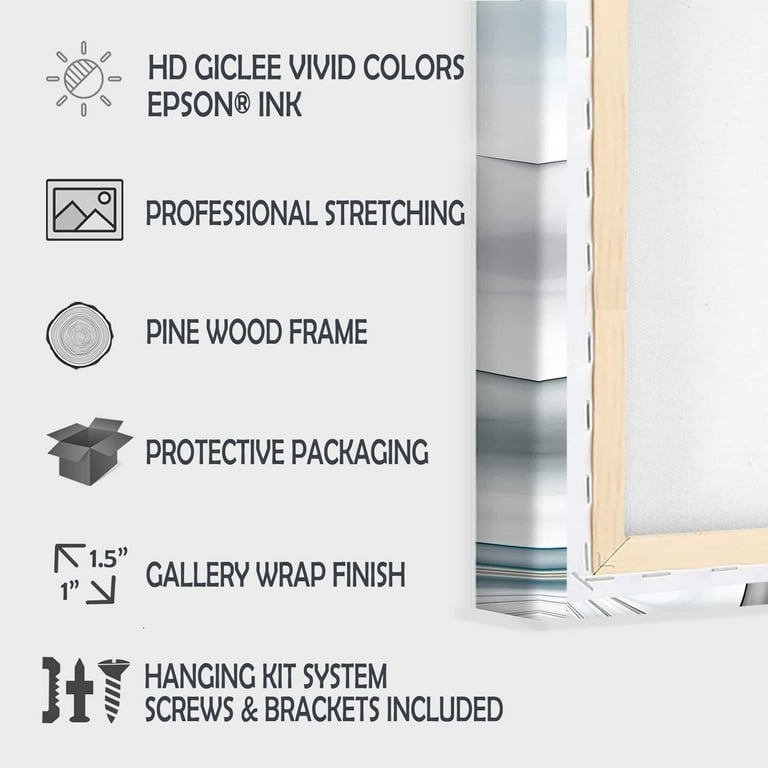This image appears to be an advertisement for a canvas printing service, showcasing various features of a canvas picture frame. The right side of the image reveals the backside of a canvas frame, complete with visible staples and stretching details, indicating that the canvas has been professionally wrapped around a pinewood frame. Some portions of the canvas show light stripes in grays, greens, and a hint of purple, though the main picture is not visible.

The left side of the image displays several icons with corresponding text detailing the product's features: 

1. A sunlight-like icon representing "HD Geigli Vivid Colors Epson Inc."
2. A photo frame and mountain peaks icon indicating "Professional Stretching."
3. A cross-section of a tree stump representing a "Pinewood Frame."
4. An open box icon signifying "Protective Packaging."
5. Two arrows indicating 1 inch and 1.5 inch for the "Gallery Wrap Finish."
6. A tools and nails icon labeled "Hanging Kit System, Screws and Brackets Included."

This comprehensive representation, along with the included hanging kit, suggests that the product is ready for immediate display. The overall setup and presentation indicate that the advertisement is aimed at customers shopping for high-quality, ready-to-hang canvas pictures in a store.